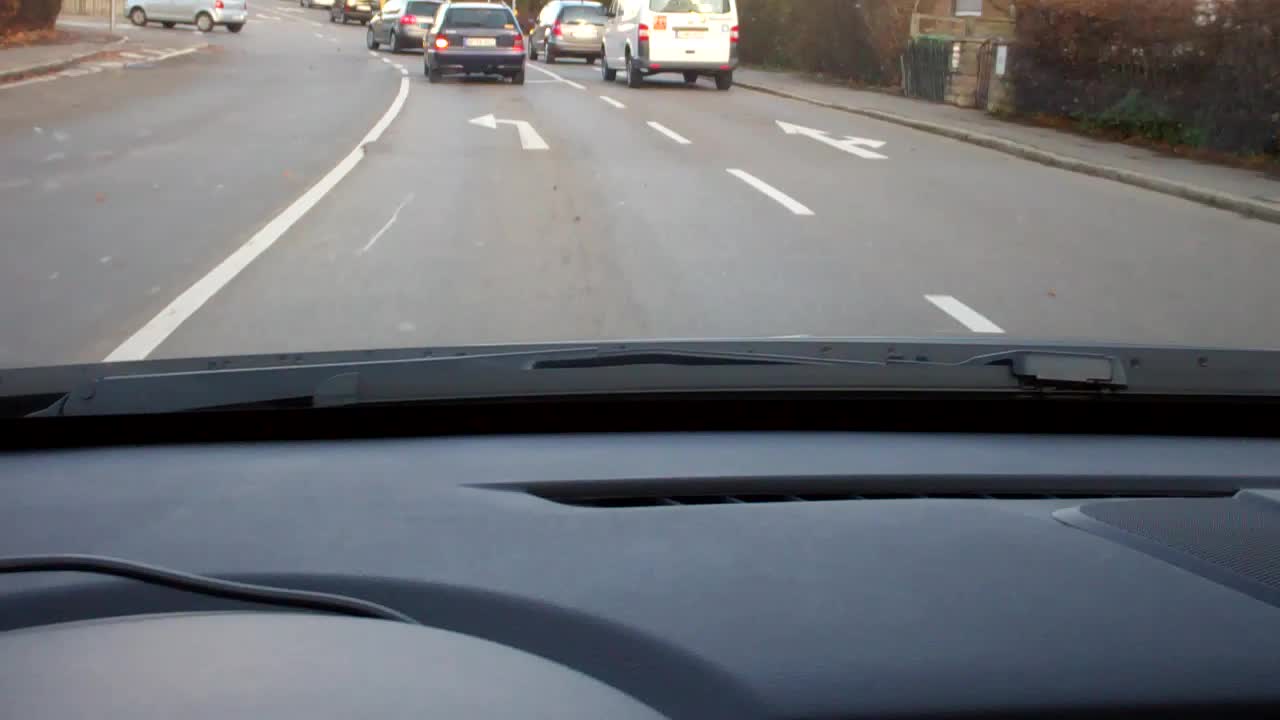The image is a detailed view from the dashboard of a moving vehicle, capturing both the interior and the road ahead. Prominently featured in the foreground are the top of the dashboard, the steering wheel section, and a visible windshield wiper. Through the windshield, an urban scene unfolds with multiple traffic lanes and marked arrows. The lane directly ahead has an arrow indicating a left turn, while the adjacent lane to the right has a dual-headed arrow pointing straight and to the right. Several cars are in view, spaced thoughtfully across the lanes; a black or dark blue sedan is a few car lengths ahead in the same lane, with additional vehicles to the right, some with brake lights and turn signals active. A silver car can be seen in the distant left lane, turning left. The road is medium grey with distinct white lane markings. Buildings with shrubs and sidewalks border both sides of this urban street, contributing to the bustling, organized road scene.